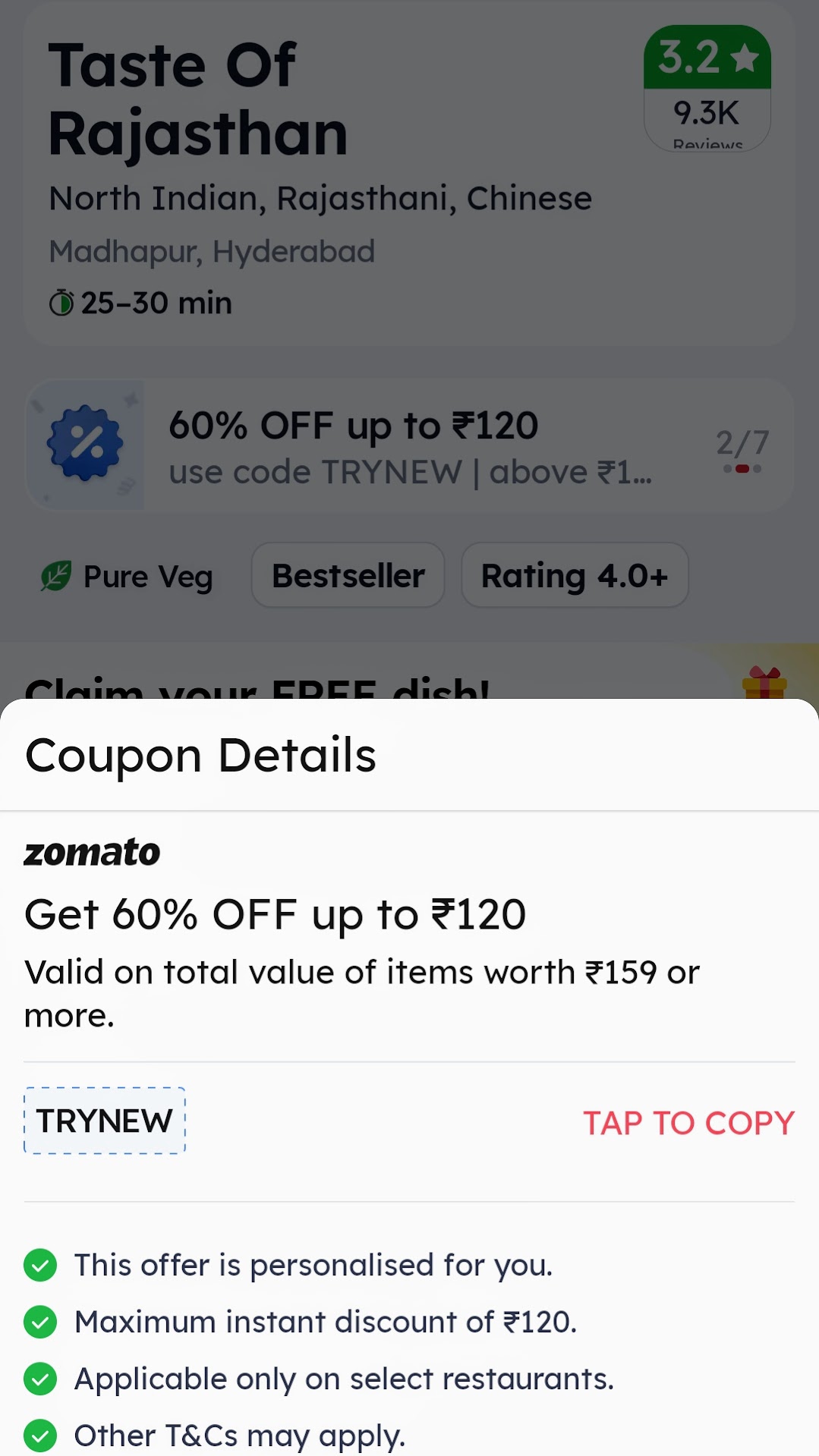The image features a promotional offer from a restaurant named "Taste of Rajasthan," which specializes in North Indian, Rajasthani, and Chinese cuisine. The restaurant has a rating of 3.2 stars (out of an unspecified total) and is currently offering a generous 60% discount on orders up to ₹120, with a promotional code "TRYNEW." Below this offer, there is an option to claim a free dish.

In the foreground of the image, a pop-up screen from Zomato provides detailed coupon information. The Zomato pop-up highlights that the 60% discount is valid on orders worth ₹159 or more. The code "TRYNEW" has been entered into a designated field with a convenient "Tap to Copy" button adjacent to it for easy use. Below this, additional terms and conditions for utilizing the coupon are listed.